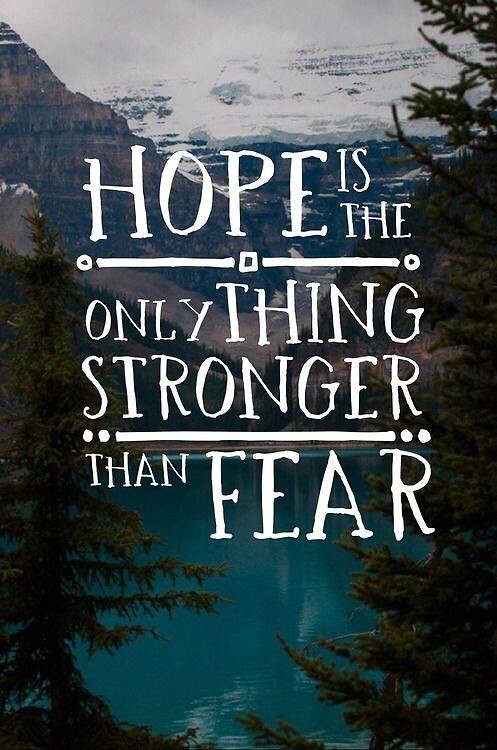The poster presents a striking evening scene in a mountain valley, evoking a sense of tranquility and hope. The background showcases a clear, light blue lake cradled between tall pine trees and leading the eye towards towering, steep, rocky mountains on the left and a snowy mountain range in the distance. The sky is dotted with different clouds, adding to the serene atmosphere. The overall tones of black and blue suggest the calmness of evening. Central to this image, in a playful, white font, are the words “HOPE IS THE ONLY THING STRONGER THAN FEAR,” a powerful and uplifting message that enhances the inspirational nature of the poster. The dark filter over the photo emphasizes the peaceful and contemplative mood, making the poster as visually stunning as it is motivational.